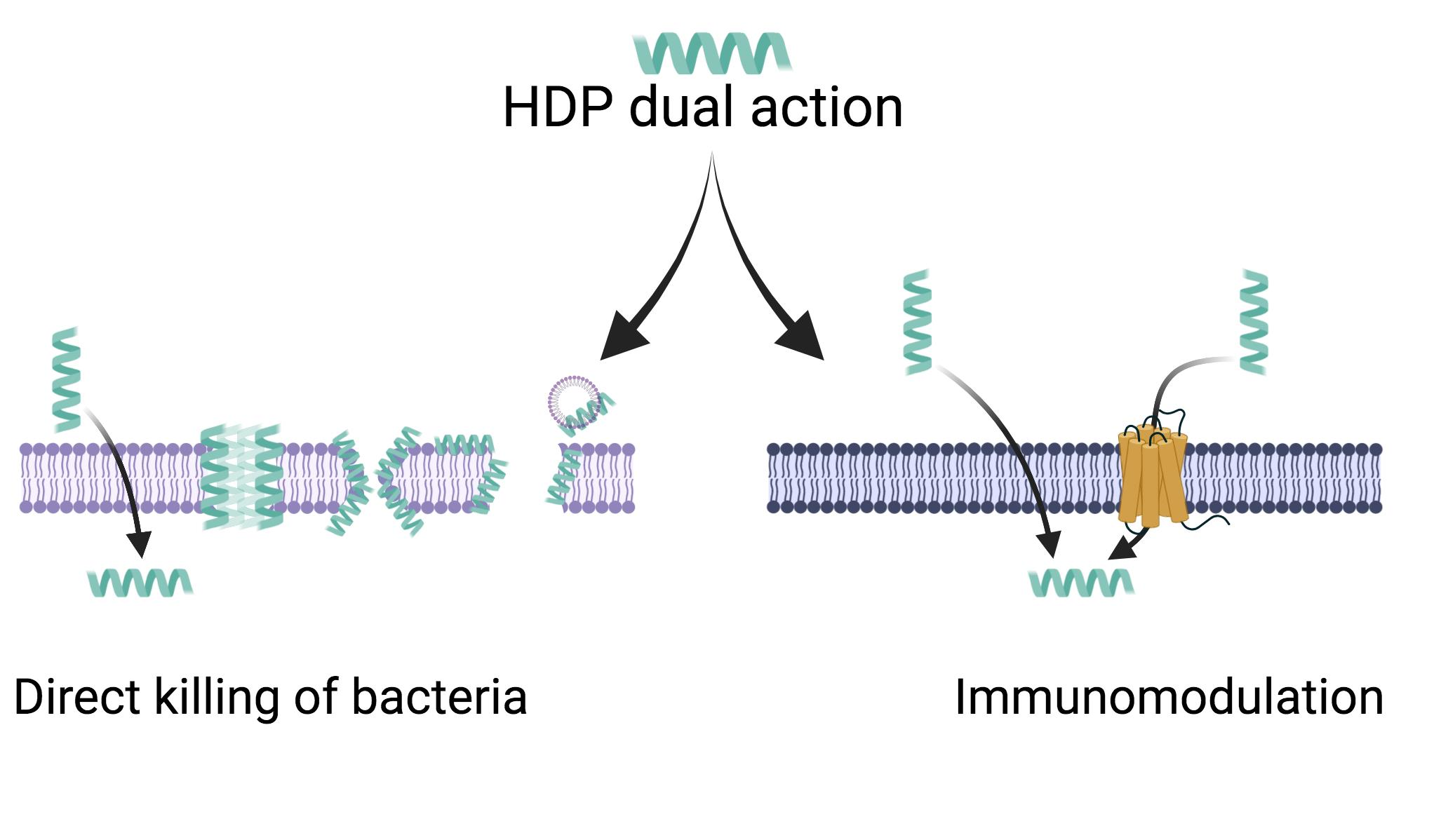This colored scientific diagram, set against a plain white background and titled "HDP Dual Action" in black font at the top center, illustrates two distinct mechanisms. Above the title is a horizontal green spiral tube. Two black, curved arrows emanate from the title—one pointing to the bottom left and the other to the bottom right. 

The bottom left section, labeled "Direct Killing of Bacteria," features a purplish tube intersected by green spiral lines at various points, suggesting the mechanism of direct bacteria eradication. 

The bottom right section, labeled "Immunomodulation," displays interconnected blue molecules, with green tubes on the exterior pointing towards an orangish-yellow central blob, indicating the immunomodulatory action.